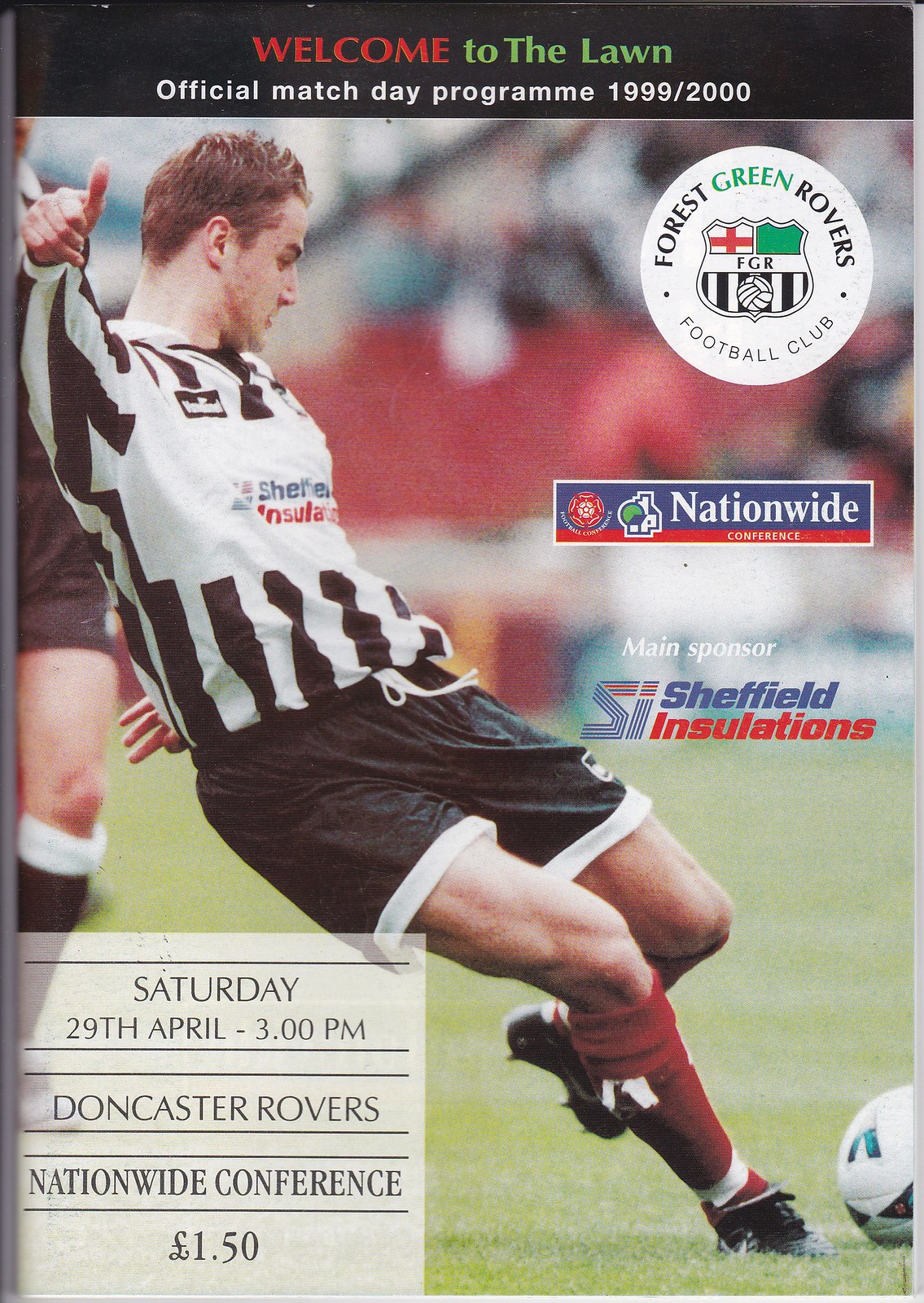The image depicts the cover of an official match day program from the 1999-2000 season, titled "Welcome to the Lawn" in colorful letters at the top. Below that, it reads "Official Match Day Program, 1999/2000" in white font. The central image showcases a soccer player dressed in a white shirt with black stripes and black shorts, in the midst of kicking a soccer ball. 

On the top right, there's a white circle bearing the name "Forest Green Rovers FGR Football Club," with "Green" highlighted in green font. Beneath this circle, a blue box with white text reads "Nationwide Conference," followed by another line in white font stating "Main Sponsor," with "Sheffield Installations" detailed below in blue and red font respectively. 

In the bottom left corner, in a black font within a box, it notes the match details: "Saturday, 29th April, 3 p.m. Doncaster Rovers Nationwide Conference." The program price is listed as £1.50.